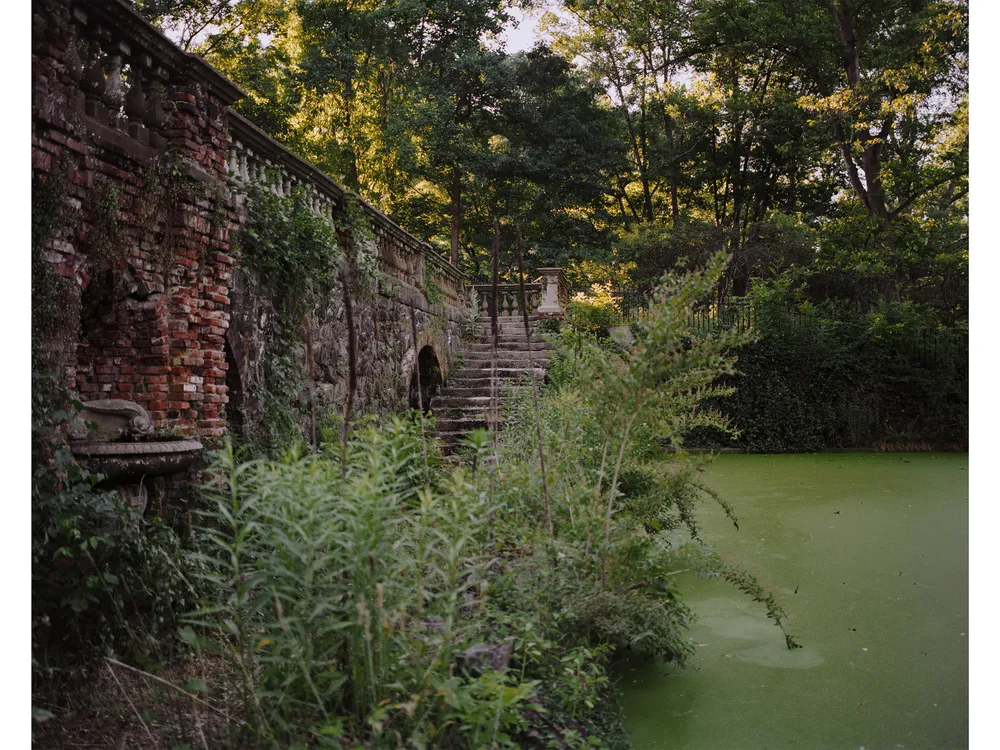The image captures a rundown, overgrown sewer area with a brick walkway alongside a stagnant, algae-filled waterway. The bricks of the walkway are a dark red, some overlaid with white moss, indicating age and wear. Concrete steps lead down to the sewer entrance, framed by dense fern foliage that suggests the abundance of summer growth. On the left, an orange and red brick wall supports a railing with white concrete posts, topped by a large, empty white planter. The scene also features tall grasses and wildflowers around the steps, contributing to the site's overgrowth. The backdrop comprises a mix of green and yellow-tinged trees, with patches of bright but dimming sky visible through the foliage, reinforcing a slightly darkening, serene atmosphere.